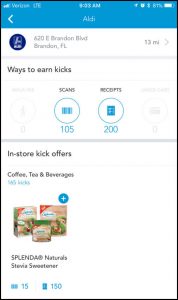**Image Description: Smartphone Screen Displaying a Shopping Rewards App**

This small, blurry image appears to be a screenshot of a smartphone, likely captured from an app under the category of Websites. The phone screen shows various indicators and app details: 

- **Top Status Bar**: 
   - The time reads either 9:03 or 8:08 AM.
   - The carrier is Verizon with LTE connectivity.
   - The battery icon indicates a full charge.
   - An alarm clock is set, and Bluetooth is enabled.

- **Address Display**: 
   - The screen features an address: 620 Brandon Blvd, Brandon, Florida, with a distance marker of 13 miles.

- **Rewards Information**: 
   - The app seems to be related to a shopping rewards system.
   - It mentions, "ways to earn kicks," where "kicks" likely refers to points or rewards within the app.
   - Various methods to earn "kicks" are displayed:
     - **Scans**: Demonstrates a barcode and lists "105 receipts" with an accompanying receipt icon showing "200".
     - **Additional Sections**: 
       - Two other circles are blurred out, indicating no active offers.
     - **In-Store Kick Offers**: Categories include items such as "coffee, tea, and beverages."
       - There is a mention of "Splenda, Naturals, Stevia, Sweetener," which offers 150 kicks.
     - There's a plus sign suggesting additional categories or offers not identifiable due to the blur.

The image suggests the user is using a shopping rewards app that offers points (kicks) for various activities such as scanning items or receipts and purchasing specific products.